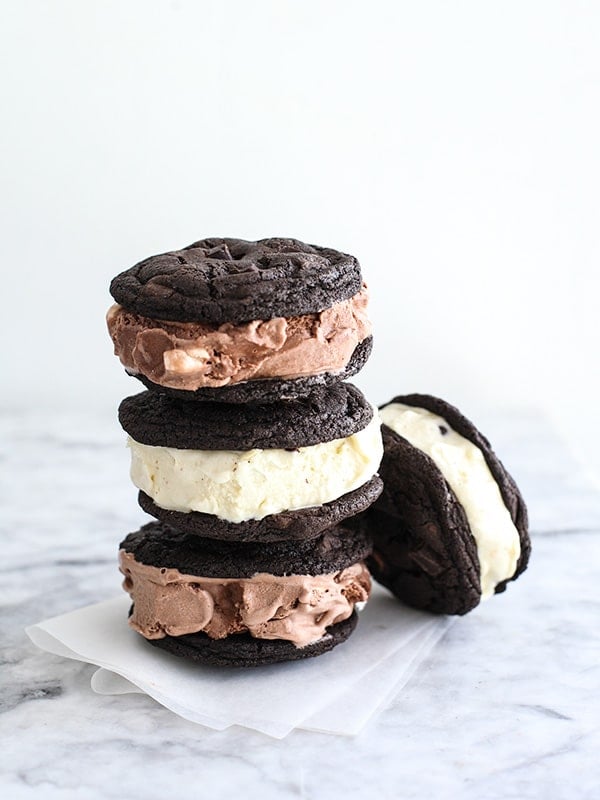A close-up photograph showcases four decadent homemade ice cream sandwiches, meticulously arranged on a folded piece of white parchment paper atop a sophisticated white and gray marble countertop. Each sandwich features a pair of rich, dark double chocolate chip cookies enveloping generous scoops of ice cream. The topmost sandwich boasts creamy chocolate ice cream, followed by a vanilla-filled creation, and another with chocolate ice cream. Leaning against this neatly stacked trio is a fourth sandwich, distinguishably filled with vanilla ice cream. The pristine white background adds a touch of elegance, accentuating the delectable contrast of deep brown cookies and creamy ice creams, making a visually tempting treat.